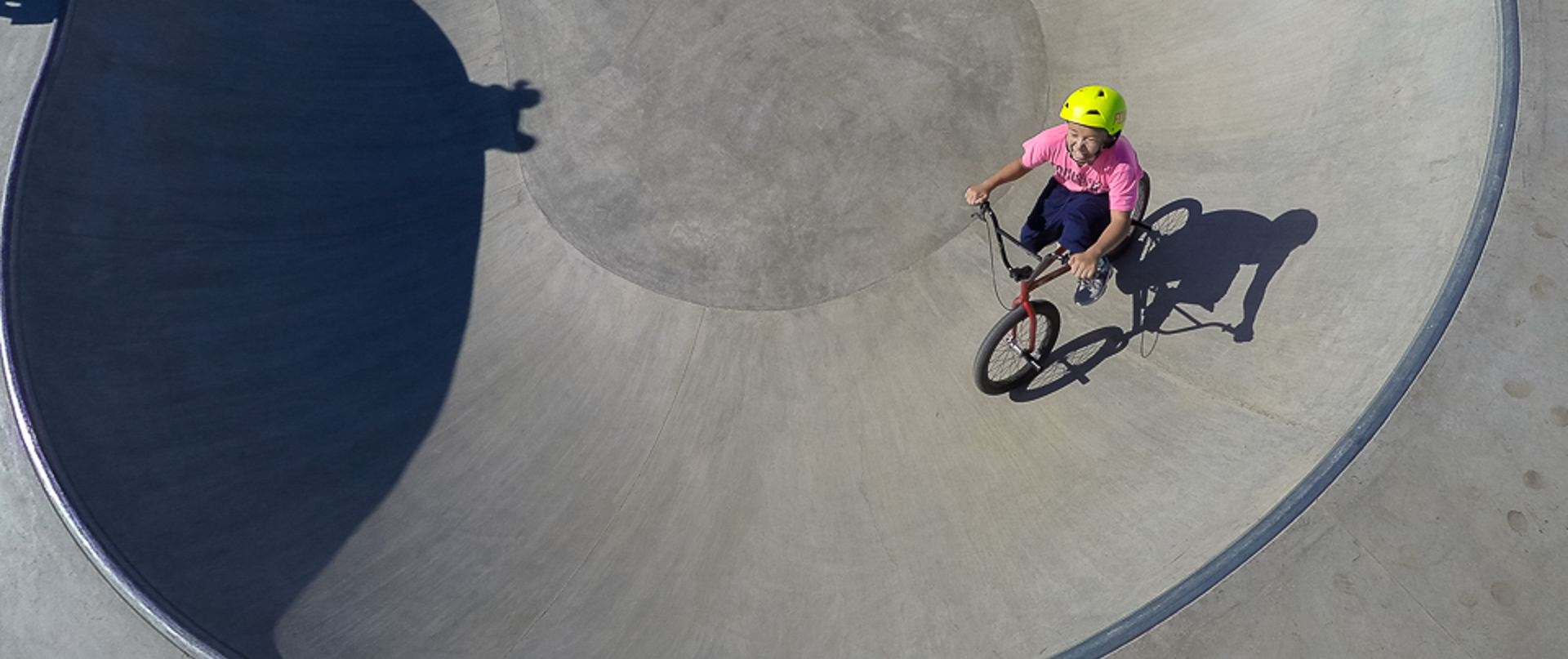An aerial photograph captures a vibrant scene at an outdoor recreational area, likely a skate park, on a sunny day. The image centers on a young child, no older than ten, riding a red BMX-style bicycle with black handlebars and peg stands on both wheels, ideal for tricks. The child, who has dark skin, is wearing a bright neon green helmet, a pink shirt, blue sweatpants, and sneakers, and appears to be smiling with their eyes closed, possibly squinting in the sunlight. They are riding within a large, gray, cement bowl that has a metal ring around the edge, designed for grinding. The bowl's shape is akin to a cereal bowl, with an upper flat area that curves inward. The intricate shadows cast by the child and their bicycle onto the concrete surface emphasize the sunny, clear day.